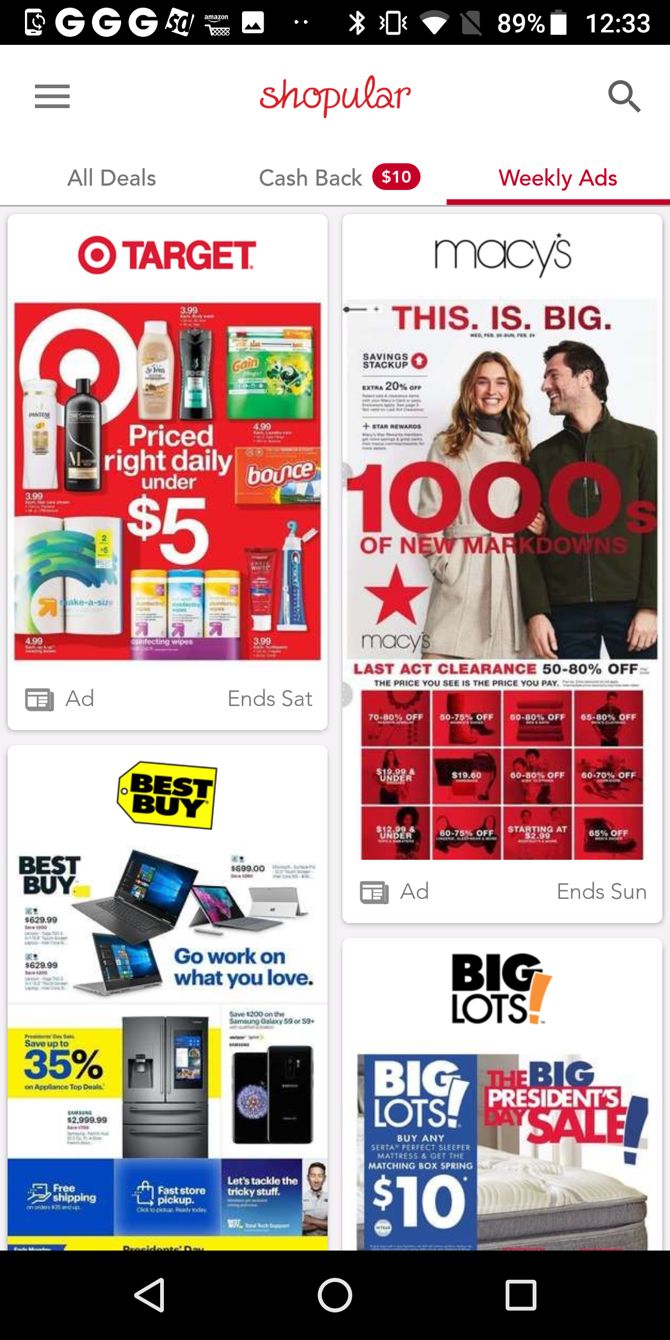This image displays a cell phone screen showcasing the Shopular app interface at 12:33 PM with an 89% battery charge. The app highlights various promotional deals and cashback offers. The top section of the screen lists categories such as "All Deals" and "Cashback," and prominently features weekly ads from popular retail stores including Target, Macy's, Best Buy, and Big Lots. 

The Target ad promotes "Priced Right Daily Under $5" deals. Macy's emphasizes "This is Big: 1000's of New Markdowns." Best Buy offers up to "35% off on Appliances," encouraging customers to "Work on What You Love." Big Lots highlights a spring promotion with a "$10 Match" and advertises the "Big President's Day Sale."

The colorful interface includes a variety of hues such as red, white, yellow, blue, orange, green, gold, purple, black, and more, making the app visually engaging and easy to navigate through different offers and advertisements.